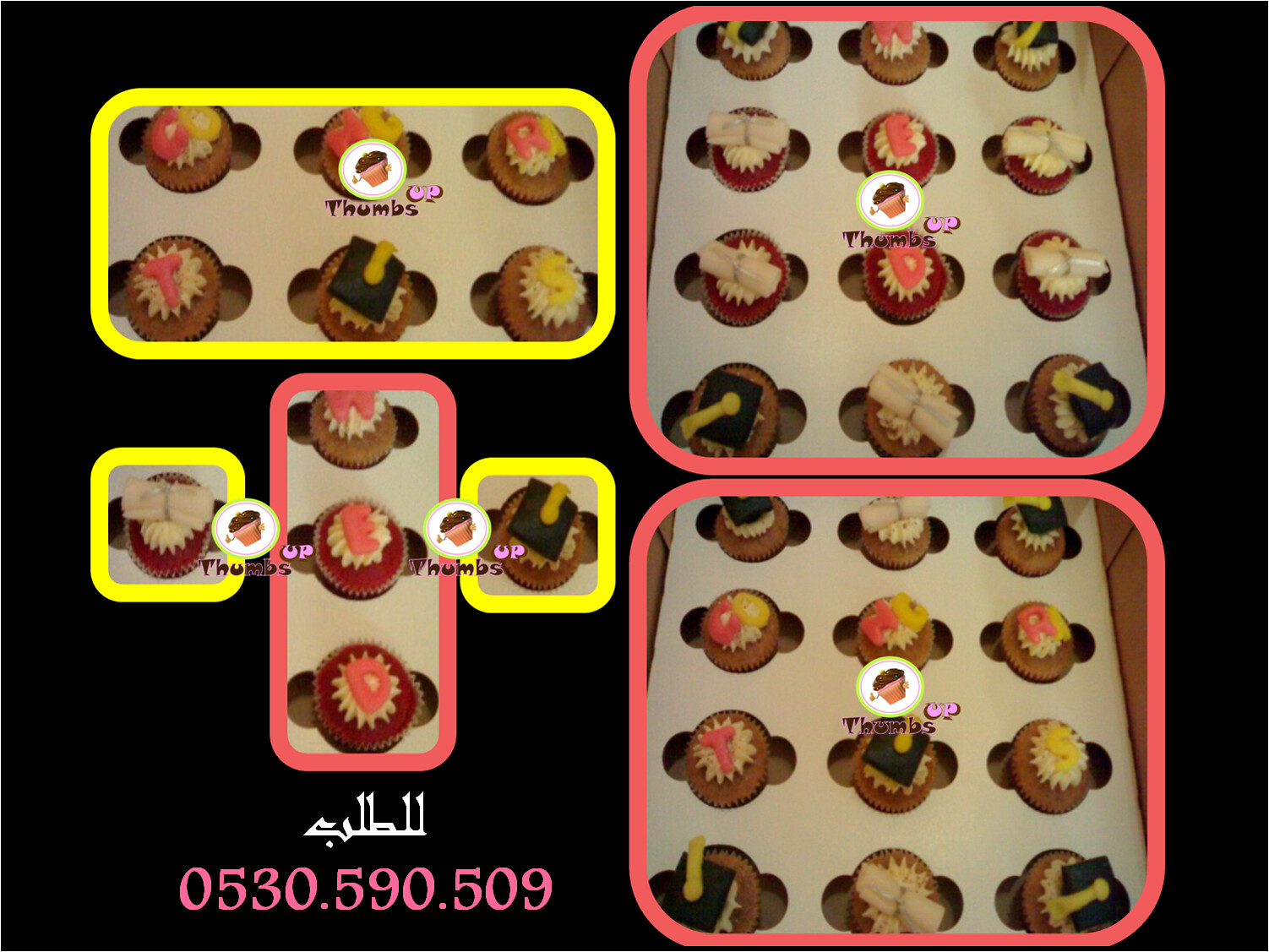The image displays a vibrant advertisement set against a black background, reminiscent of a video game interface. Centered in the composition, a prominent yellow rectangle contains two rows of three intricately decorated cupcakes, each with distinct frosting designs, some even adorned with graduation hats. Flanking this centerpiece to the right, a large pink rectangle houses a grid of twelve cupcakes arranged in four rows and three columns. Directly beneath it, another identical pink rectangle holds the same grid formation of cupcakes.

To the left of the central yellow rectangle, two single yellow squares each enclose an individual cupcake, both displaying unique frosting. Between these yellow squares is a vertical pink rectangle containing a single column of three cupcakes. At the upper left corner, there’s a rectangle surrounded by a yellow border holding three rows and two columns of cupcakes, each styled with a variety of toppings.

The cupcakes are all consistently displayed in crinkly paper cups. Below the vibrant displays, the number 0530.590.509 appears in pink font, suggesting a contact or promotional detail, accompanied by indistinct white text that possibly offers additional information. The entire scene is connected with bright, solid color trims, creating a cohesive and eye-catching layout designed to attract attention.